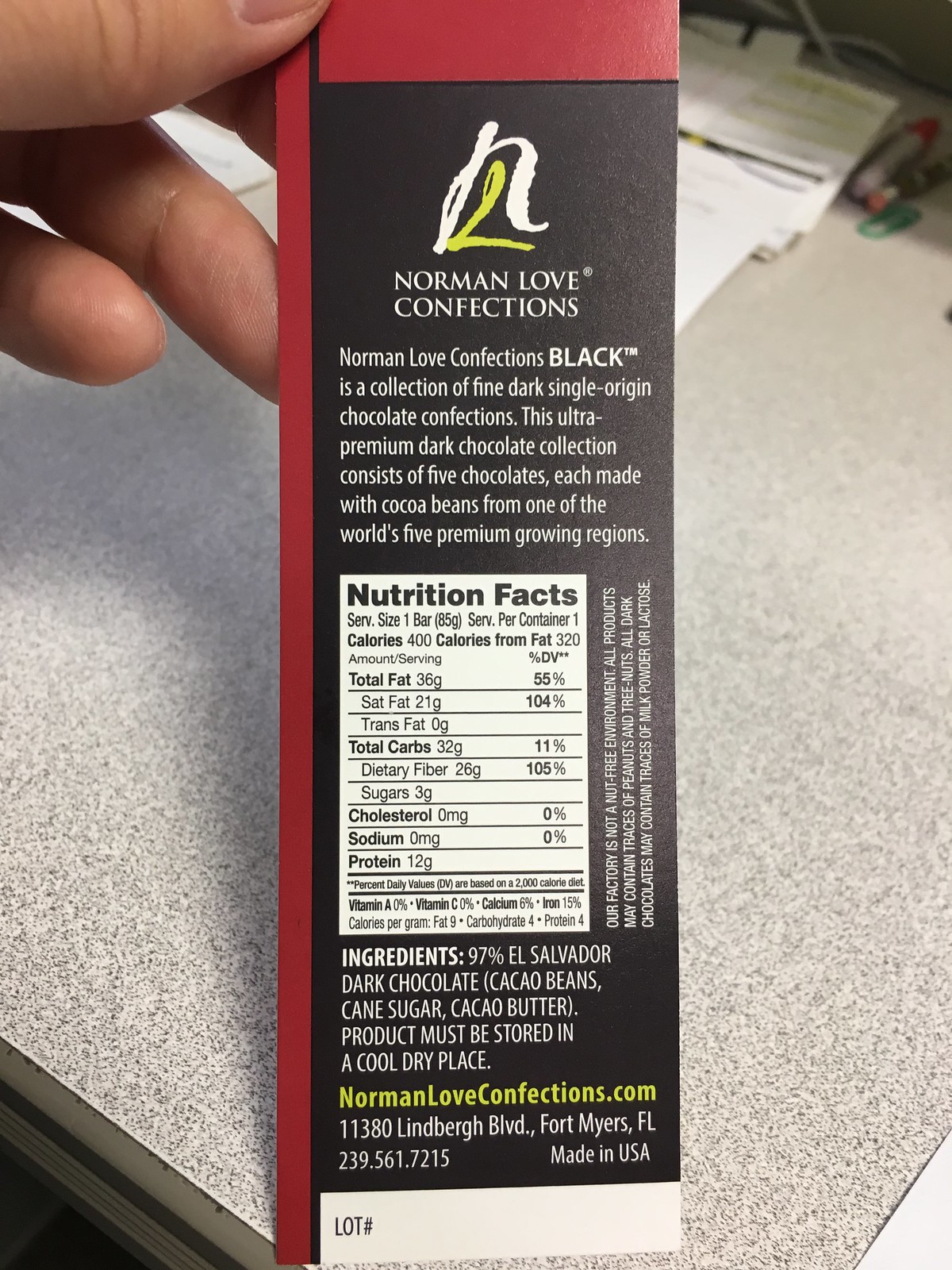In the photograph, a hand is holding the packaging of a Norman Love Confections chocolate bar, focusing on its ingredient and nutrition panel. The packaging is constructed from cardboard and features a distinctive red trim. The background of the image is predominantly black, highlighting the white and yellow logo prominently displayed at the top. Just below the logo, the text "Norman Love Confections" is clearly marked in white. The packaging describes Norman Love Confections Black as an exclusive collection of fine dark chocolate confections, made with single-origin cocoa beans sourced from five of the world's top cocoa-growing regions. Further down, a white label marked "Nutrition Facts" in black font provides detailed nutritional information, followed by a list of ingredients and the URL "NormanLoveConfections.com" highlighted in yellow. The chocolate bar packaging is held over a desk, with various papers and pens scattered in the background, adding context to the setting.